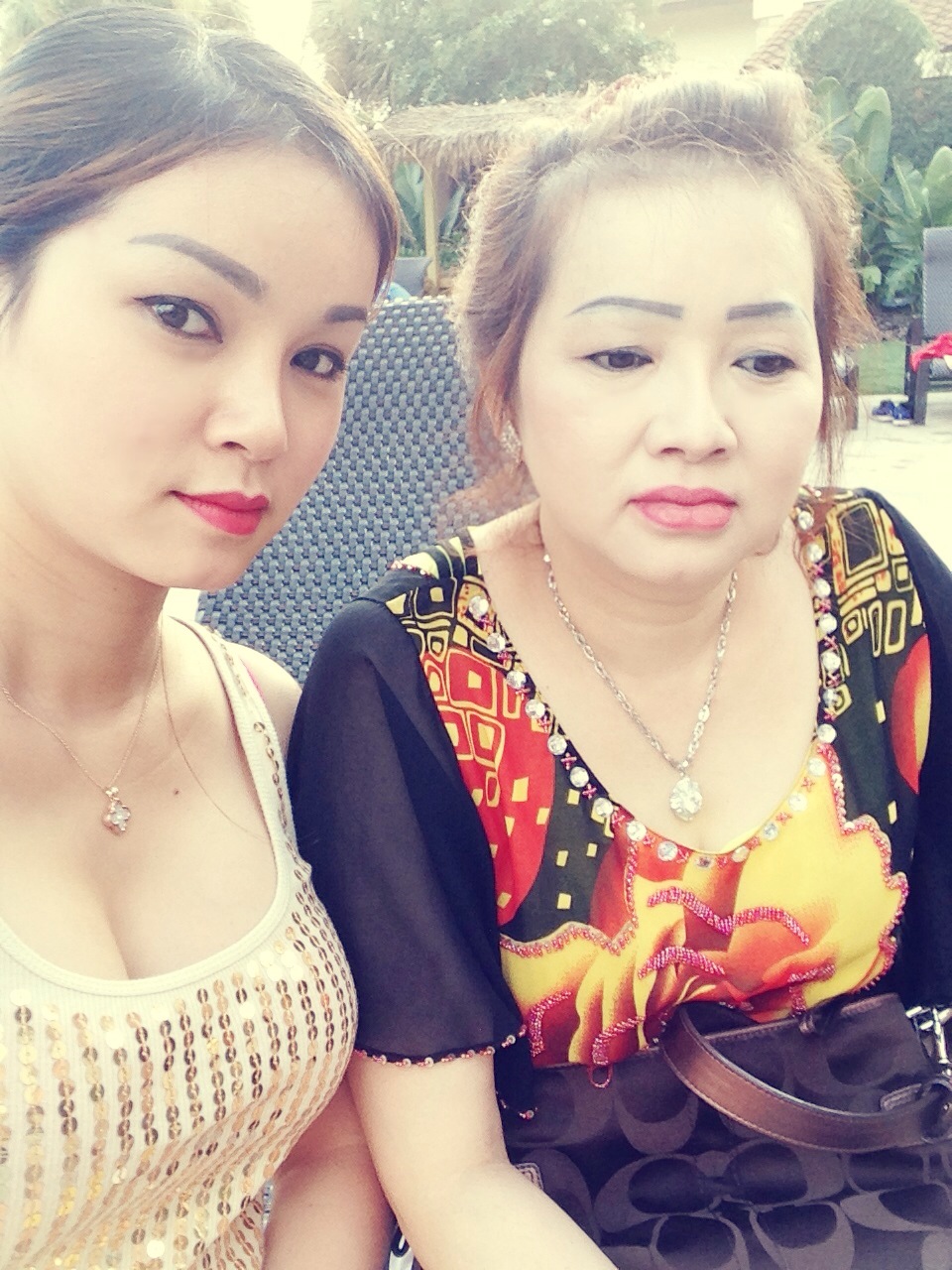This photograph, taken in portrait orientation on a sunny day, features a mother and daughter of Asian descent as the main subjects, seated closely together with tropical plants and palm trees in the background. Both women, adorned with carefully applied makeup and striking red lipstick, have their hair pulled back with subtle reddish highlights, showcasing their well-groomed eyebrows. 

The mother, positioned on the right, wears a black short-sleeve top decorated with reddish-orange flowers and holds a black bag on her lap. Her silver pendant rests elegantly against her neckline. The daughter, sitting on the left and making direct eye contact with the camera, sports a sparkly cream-colored tank top. Her necklace features a diamond-colored pendant with a gold band, complementing her dark pink lipstick and pronounced eyeliner. 

Their close placement and relaxed poses underscore the bond between them, while the lush green tropical plants in the background add a serene and vibrant touch to the overall composition.